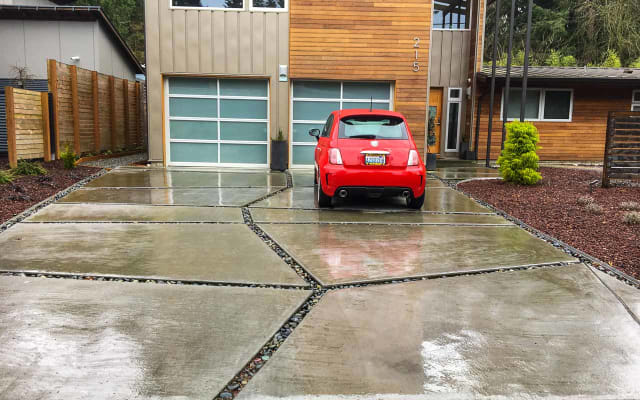This image captures a rainy day scene in front of a two-story residence with a wooden exterior and wood slats. Central to the image is a concrete block driveway, bordered with reddish gravel, leading to a two-car garage with closed doors. A red sedan is parked in front of the right garage door. The house, marked with a white number "215," features a section that juts out at a 90-degree angle above the garage. In the foreground, a small bush and a little tree are planted in mulch near the house. A wooden fence lines the left side of the driveway, and the background is filled with lush green trees.